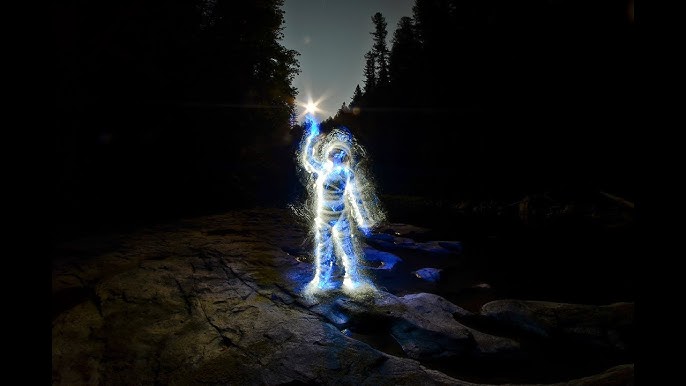The image features a striking, futuristic nighttime scene set in a small clearing within a dense forest. At the center stands a humanoid figure composed entirely of radiant light, their form outlined in blue and white hues resembling electric currents. The figure is indistinct and faceless, but the silhouette of their torso, arms, and legs is clearly visible. One arm is raised, reaching towards a bright, star-like object suspended above. The surrounding environment is shrouded in darkness with only the sky above the trees offering a dim, bluish-gray backdrop. The ground beneath the figure appears to be a rocky surface bordering a shallow, murky creek, encased by the silhouettes of tall, dense trees. The overall composition suggests a scene where the solitary illuminated figure contrasts starkly against the shadowy forest, emphasizing the ethereal and otherworldly atmosphere.